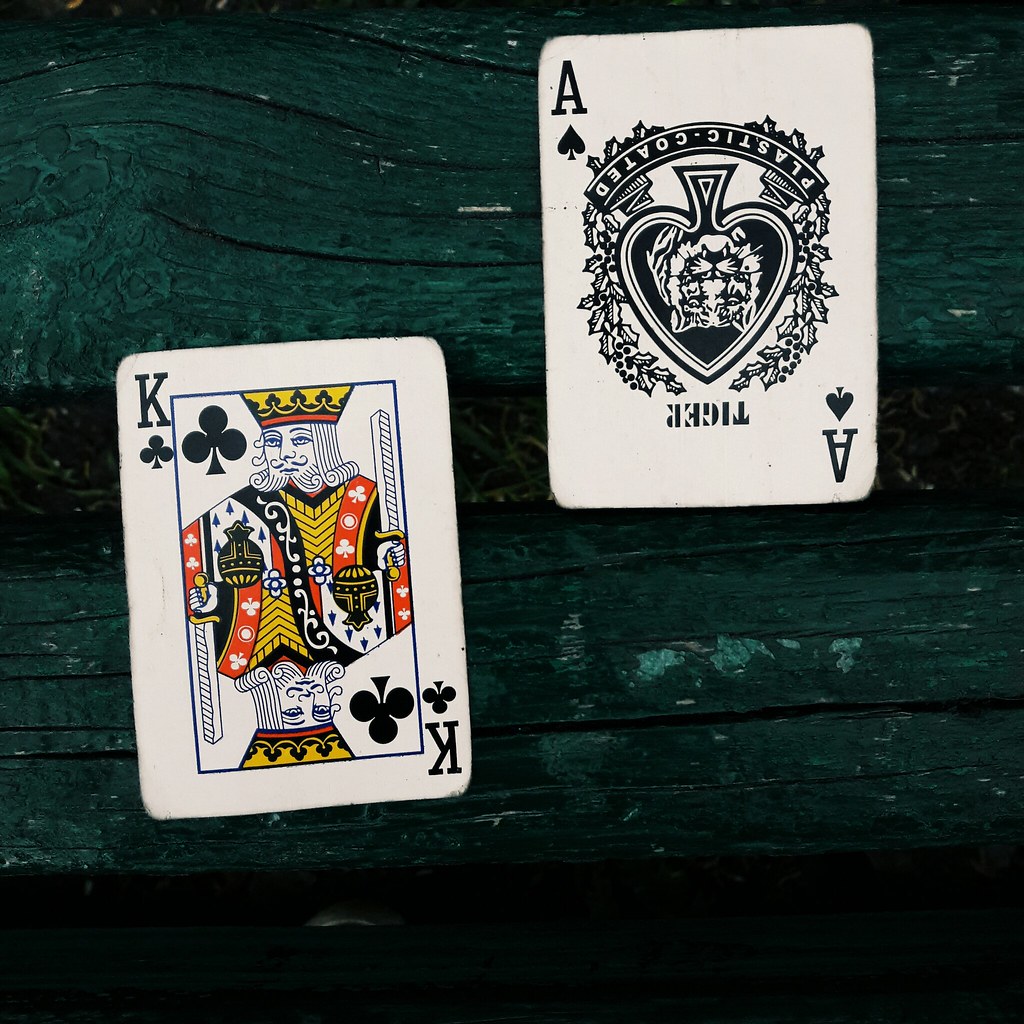Resting on a weathered, dark aqua blue wooden surface with visible grains, striations, scratches, and knots, this image captures the rustic beauty of the wood accented by patches of green grass peeking from below. The wooden boards, running horizontally across the image, each have unique marks; the top board is distinguished by white scratches and natural imperfections, while the bottom board displays significant cracks, including a prominent one stretching from right to left.

In the foreground, positioned about an inch from the left edge and centrally aligned, lies a King of Spades playing card. The card is characterized by its white border and a black frame enclosing the illustration of a traditionally attired king with a yellow crown, beard, long hair, and holding a sword in his left hand. The typical card symbols—spades—decorate both the top left and bottom right of the King’s image, with corresponding icons in each corner.

Slightly up and to the right of the King of Spades, the Ace of Spades card rests upside down. This card is adorned with a detailed illustration of a tiger's head at the center, positioned towards the bottom due to its reversed placement. Below the tiger, the word "TIGER" is emblazoned in upside-down lettering. The Ace of Spades features the spade symbol prominently in the top left and bottom right corners, accentuating the overall intricate design.

The interplay between the vivid details of the playing cards and the textured wooden backdrop creates a visually engaging composition, blending elements of classic gaming with rustic aesthetic charm.